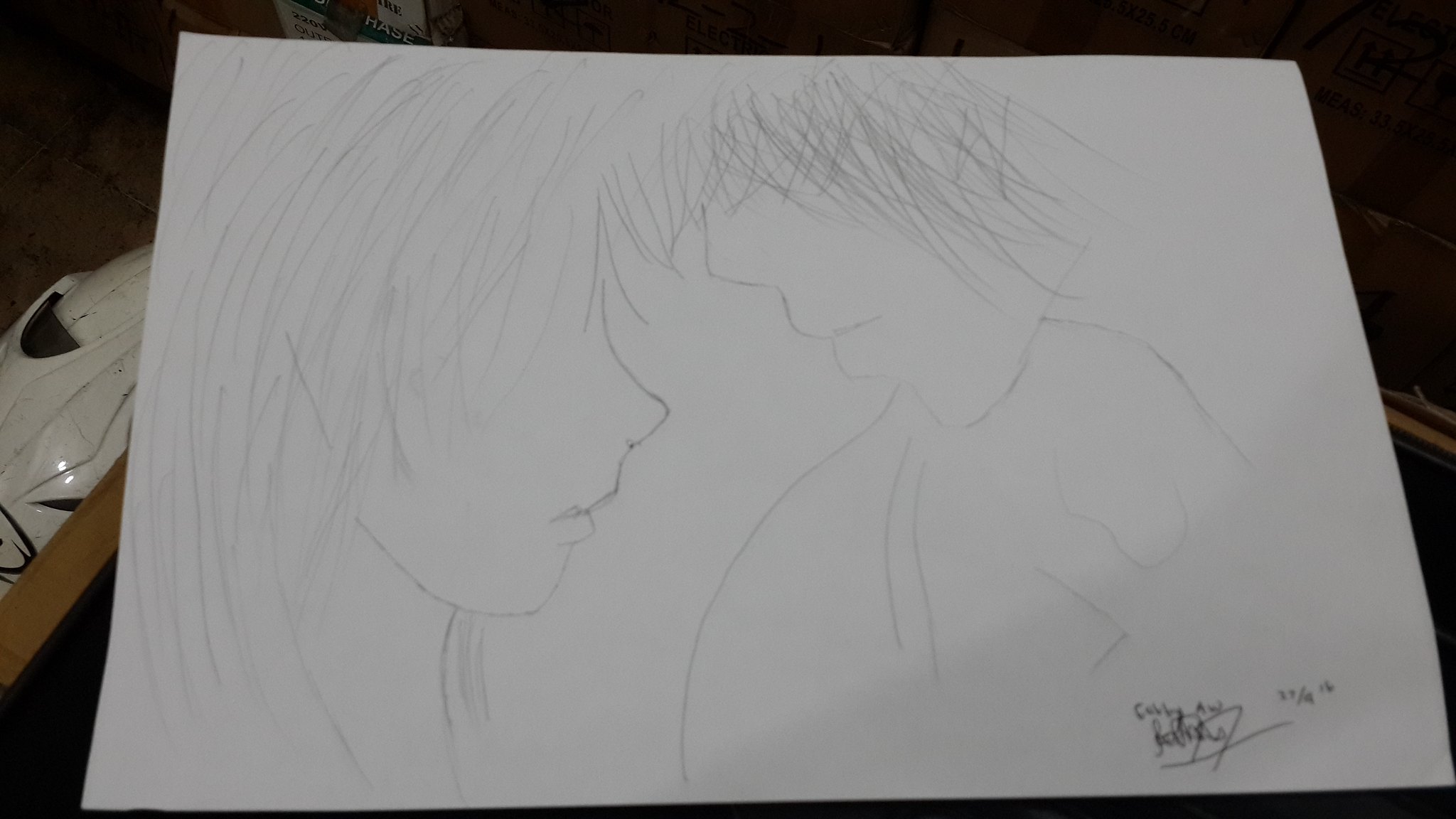This color photograph captures a detailed pencil sketch on a piece of white paper, laid on a table next to a white glove and what appears to be a striped pillow. The drawing, signed and dated November 9, 2016, in the bottom right corner, depicts a young woman and a teenage boy. The young woman is on the left side, shown in profile with her petite nose, lips, and a long neck. Her long bangs obscure her eyes. She faces a boy on the right, whose foreheads are touching. The boy, with somewhat long, shaggy hair covering his eyes, has exaggeratedly large lips and a simple, V-shaped nose. His head appears slightly tilted downwards lacking visible neck detail. Both figures seem to be intimately close, their hair mingling together subtly.